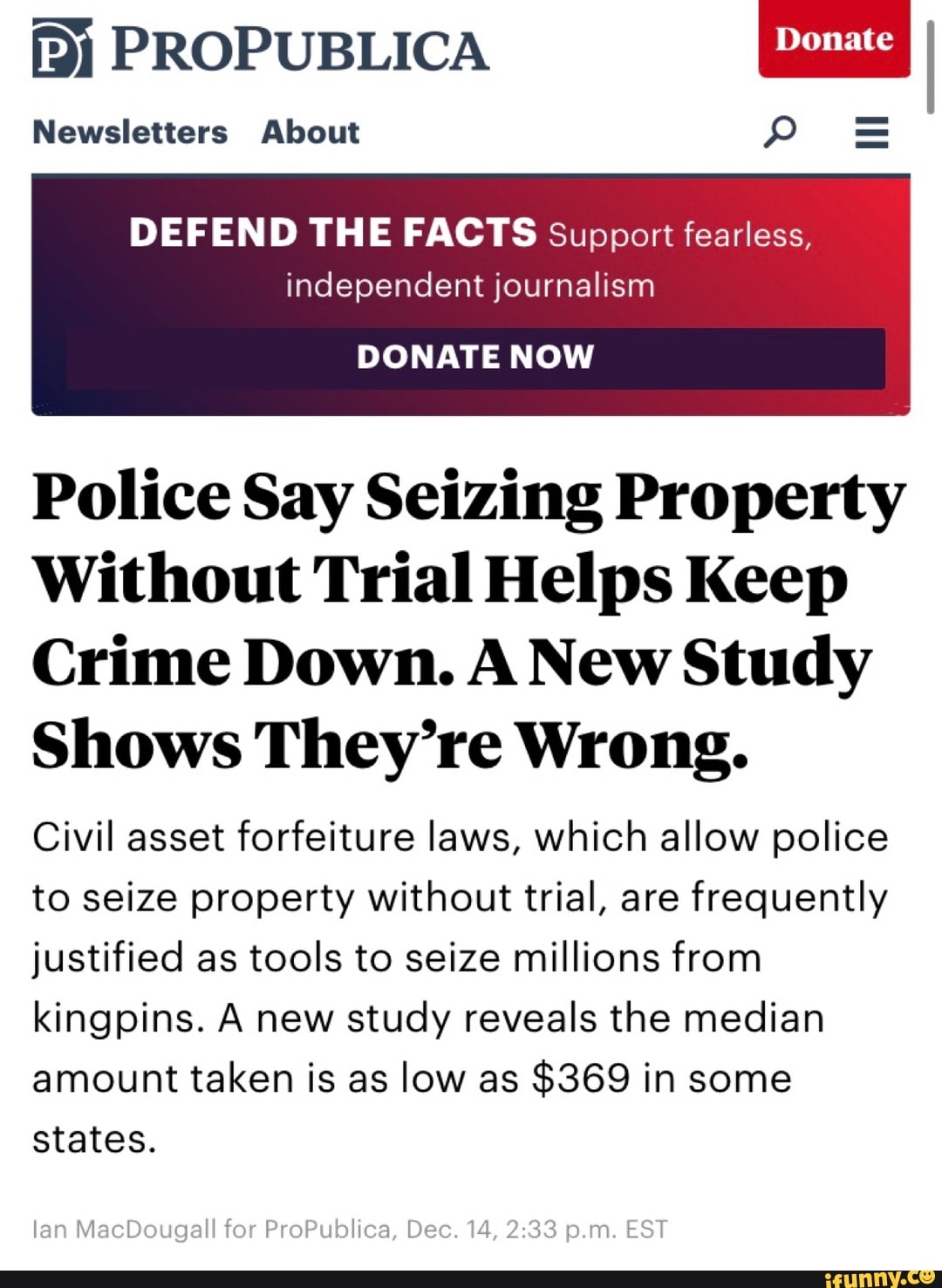This is a detailed caption for an image based on your description:

---

In the screenshot, seemingly captured on a smartphone, the ProPublica logo is prominently displayed in the upper-left corner. The logo features a "P" magnified within a square, symbolizing investigative precision. Adjacent to it in the upper-right, there is a red "Donate" button shaped like a tab extending from the top edge of the screen. Below the logo, a navigation bar presents options such as "Newsletters," "About," a magnifying glass for search, and a hamburger menu on the far right. Dominating the upper section is a gradient background transitioning from dark purple on the left to lighter red on the right. It houses a bold call to action: "Defend the facts. Support fearless, independent journalism," followed by a vivid purple "Donate Now" button in white bold letters.

Beneath this, a prominent headline reads: "Police say seizing property without trial helps keep crime down. New study shows they’re wrong." Below the headline, an explanatory synopsis highlights the issue of civil asset forfeiture laws, noting that these laws, which permit the police to seize property without trial, are often justified as a means to confiscate millions from kingpins. However, a new study reveals that the median amount seized is merely $369 in some states. The article is authored by Ian MacDougall and timestamped December 14th at 2:33 PM Eastern Time. 

At the bottom of the screenshot, a black bar spans the width. Superimposed on the image is a watermark from iFunny.co, which commonly appears on shared screenshots.

---

This caption provides a detailed and organized description of the screenshot, covering all mentioned elements and their significance.